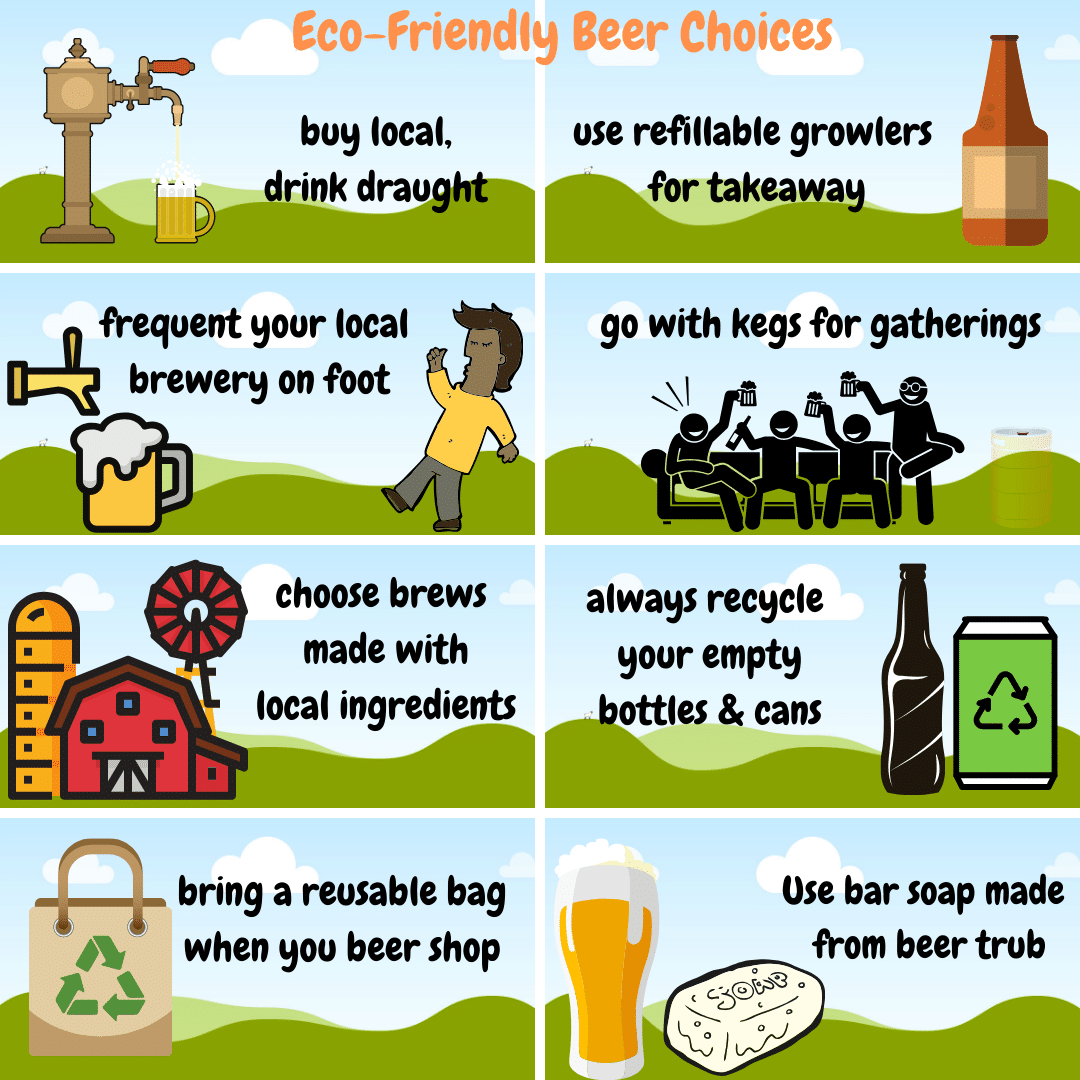This is a large square cartoon image titled "Eco-Friendly Beer Choices" in orange letters on a blue background. The image is divided into eight rectangular panels, four on the left and four on the right, each with a specific eco-friendly beer tip and corresponding illustration. 

- **Top Left:** "Buy local, drink draught" shows a spout pouring beer into a nearly full mug.
- **Top Right:** "Use refillable growlers for takeaway" features a brown bottle with a tan label.
- **Second Row Left:** "Frequent your local brewery on foot" depicts a man walking towards a foamy beer mug.
- **Second Row Right:** "Go with kegs for gatherings" displays silhouettes of four people holding beer mugs around a bench.
- **Third Row Left:** "Choose brews made with local ingredients" includes a windmill, barn, and silo.
- **Third Row Right:** "Always recycle your empty bottles and cans" shows a bottle and a recycling bin with triangular arrows.
- **Bottom Row Left:** "Bring a reusable bag when you beer shop" illustrates a bag with recycling arrows.
- **Bottom Row Right:** "Use bar soap made from beer trub" depicts a large foamy beer mug next to a bar of soap.

The consistent emphasis on eco-friendly practices is visually represented in a clear, cartoonish style throughout the image.